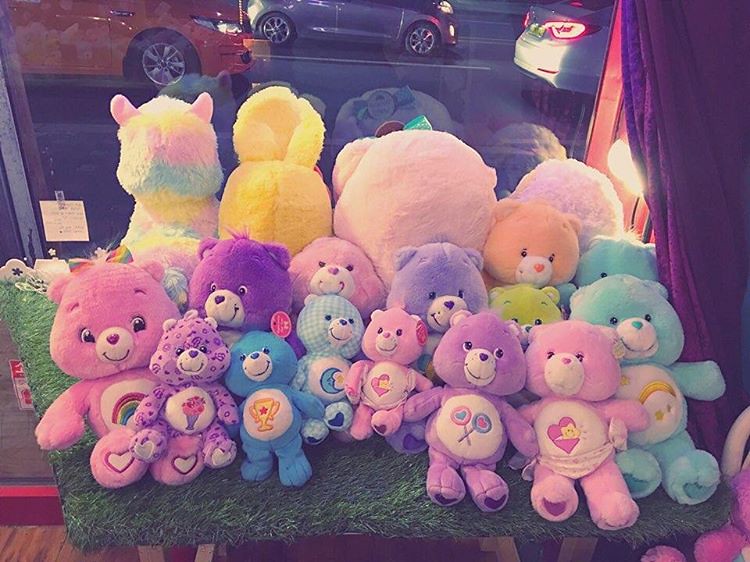A color photograph, taken in landscape mode, features an array of Care Bears and other stuffed animals meticulously arranged on a green, astroturf-covered surface. The Care Bears, numbering at least 15, come in a variety of colors including pink, blue, plaid blue, solid blue, purple, yellow, green, and peach. Each bear displays a unique embroidered symbol on its white stomach, such as a rainbow, a bouquet of flowers, a heart, lollipops, a moon, and a trophy. Their paws often sport heart patterns, a classic Care Bear trait. The stuffed animals rest in a snug, slightly leaned-back arrangement, with some in front rows and others nestled behind them.

In the background, larger stuffed animals like a rainbow-colored llama and pink, yellow, and smaller round pink circles—possibly representing sheep—are positioned with their backs facing outwards. They all look through a large window, beyond which lies a nighttime street scene featuring three cars: an orange sedan, a gray Porsche, and part of a Saturn. A purple curtain drapes to the right of the window, and an unreadable posting note is taped on the glass. The overall image has a pinkish, cloudy overlay texture, adding a whimsical feel to the storefront display.